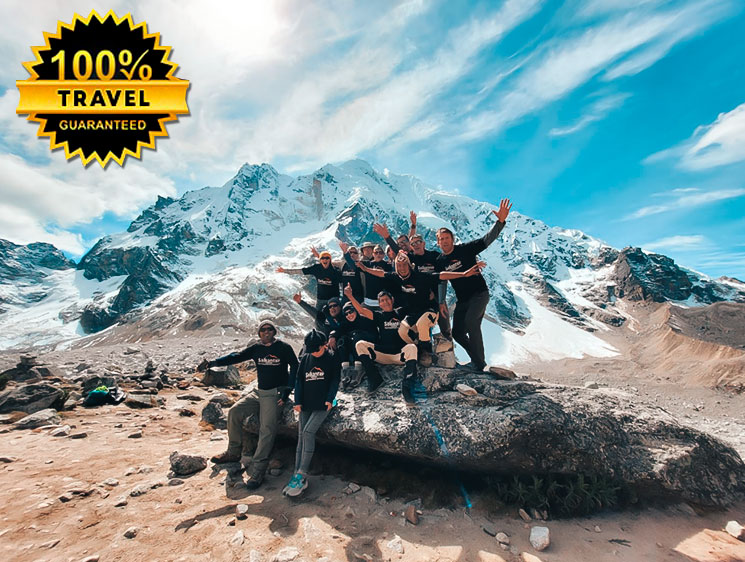This photograph captures a group of around ten to twelve enthusiastic individuals at the base of a snow-capped mountain peak. They are standing and sitting on a large, flat tree stump or rock amidst medium brown dirt and rocks, with no snow at their feet. The people are wearing a mix of long-sleeve shirts and t-shirts, some of which appear to bear a similar logo, possibly Patagonia, suggesting they are dressed for cold weather. The group is exuberantly posing for the camera with outstretched arms, waving, and one person giving a thumbs up, indicating a sense of achievement. The clear, bright blue sky above features wispy white clouds.

In the foreground, two individuals are seated on the rock: a dark-skinned man with gray pants and boots extending his arm outward, and a person next to him, possibly female, wearing a black hat and boots with bright blue laces. Behind them stand several other group members against the striking backdrop of the snowy mountain.

The upper left corner of the image contains a starburst-shaped logo with a black and yellow design. It has "100%" written above a yellow banner that says "TRAVEL" in black text, and below that, "GUARANTEED" in yellow text, suggesting that the photo might be associated with a travel promotion or magazine cover.